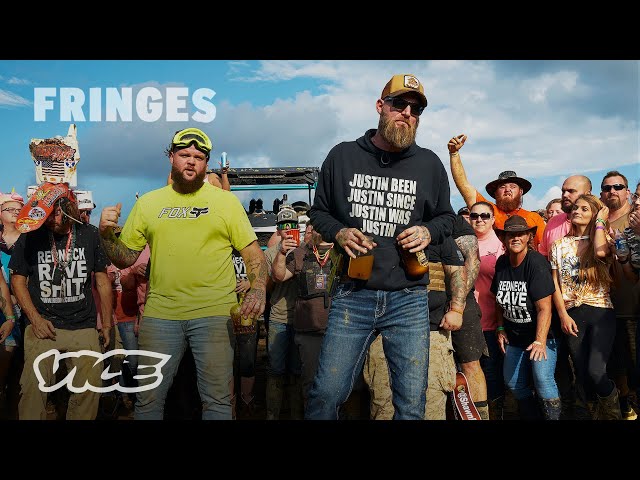The image depicts a lively crowd of people at what appears to be an outdoor event, with noticeable branding suggesting it is related to VICE Media. Both the top right corner and the bottom left corner display captions, "Fringes" and "Vice" respectively, the latter outlined in stylized letters. A diverse assembly of attendees faces the camera, many adorned in casual attire such as jeans, khakis, and various T-shirts. In the foreground, two men stand out: the one on the right wears a yellow hat and a hoodie emblazoned with the phrase "Justin been Justin since Justin was Justin," while the man on the left sports a lime-green T-shirt with the logo 'Fox' and a neon green ski mask atop his head. Both men have prominent beards. Behind them stretches a large structure that could be either a stand or the top of a stage. The crowd is animated, with some individuals—like a man raising his fist—displaying signs of merriment, and a number of attendees holding beer cans. Additional notable figures include a woman in a cowboy hat with a "Redneck Rave" T-shirt and another woman adorned with numerous bracelets. The scene suggests a festive atmosphere, possibly a concert or similar gathering, characterized by a unique cultural flair.